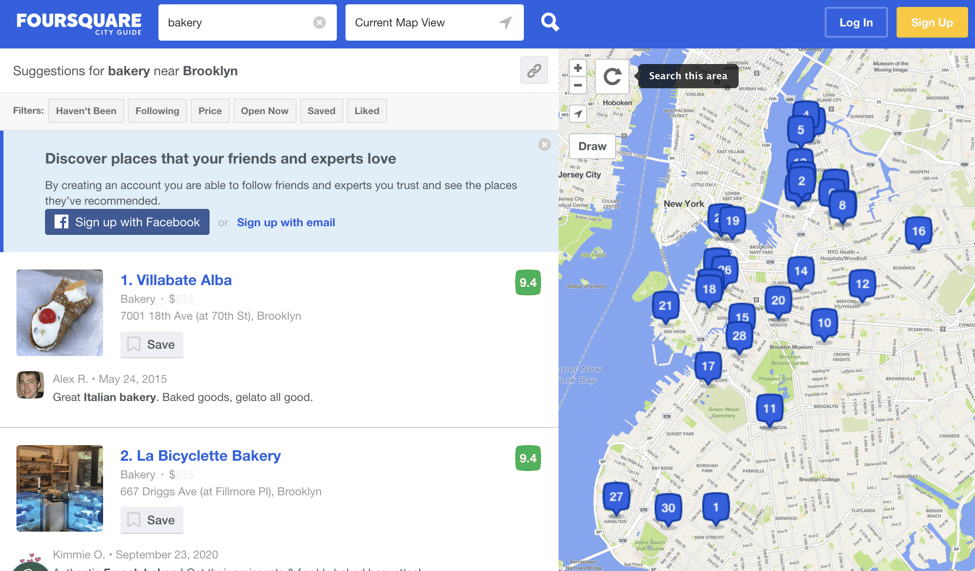This screenshot showcases the Foursquare City Guide website interface. At the top of the screenshot is a blue navigation bar, which features two primary fields: a search field on the left and a location field immediately to its right, both accompanied by a magnifying glass icon. On the far right of the bar are the login and signup buttons, with the login button in blue and the signup button in yellow.

Beneath this bar are suggestions for bakeries near Brooklyn. Following that, several filter options are presented as separate buttons, labeled "Following," "Price," "Open Now," "Saved," and "Liked."

The main section of the screenshot highlights an invitation to discover places that friends and experts recommend. Users are prompted to create an account to follow trusted recommendations, with options to sign up via Facebook or email.

Further down, two bakery suggestions are displayed: "Villa Bay Alba" and "Love Bicycle." To the right is a map showing approximately 30 bakery suggestions throughout Brooklyn, New York. The map features interactive elements including plus (+) and minus (-) buttons for zooming, an arrow pointing to the top right, a draw button beneath the arrow, and a search area button to the right of the zoom controls.